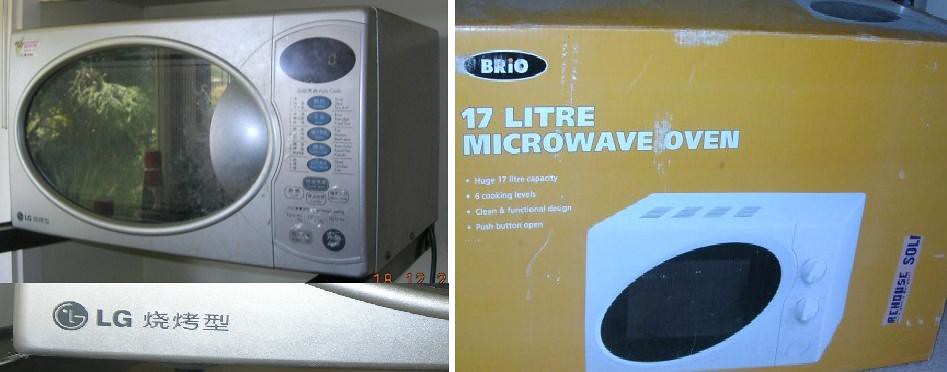The image is composed of two photographs side by side. On the left, there is a silver LG microwave oven with a round see-through glass door. The controls, which are circular and vary in size, are positioned to the right of the door. Above the touch panel, there is a dark oval display showing a lit-up zero. The bottom right corner of this half contains a timestamp from a camera, displaying the numbers 18, 12, and 2. Beneath the microwave image, there is a close-up of the bottom left corner, showing the LG brand logo along with some Chinese characters.

On the right side of the image is the box that the microwave came in. The box is orange and prominently features the brand name BRIO, written in white letters within a black oval at the top left. The box describes the microwave as having a "huge 17-liter capacity," "six cooking levels," "clean and functional design," and a "push button open." The microwave pictured on the box is white, with a darker, angled circular see-through door and knobs on the right.

This photograph appears to be taken to showcase the microwave and its packaging, possibly for sale purposes.